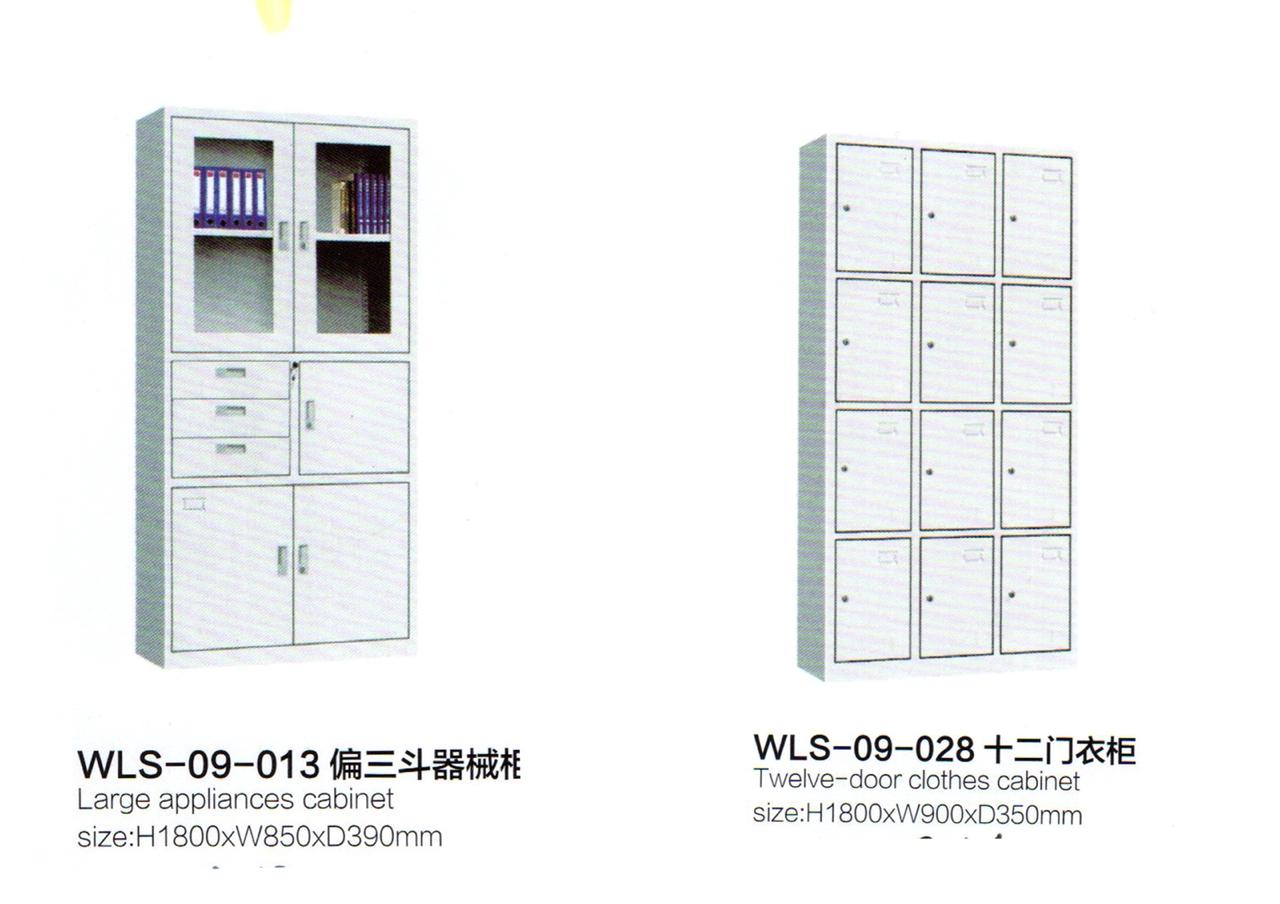The image appears to be a catalog page showcasing two detailed AI-rendered cabinets. On the left, there is a white cabinet labeled with the code WLS-09-013 followed by some Chinese or Japanese characters. This large appliances cabinet has dimensions of H1800 x W850 x D390 millimeters. The cabinet features a versatile design with various compartments: two glass cupboard doors at the top, displaying what seem to be blue notebooks, a white binder, and some blue and goldish-black books. Below the glass doors are three pull-out drawers on the left and a smaller cupboard door on the right. At the bottom, the cabinet has two additional smaller cupboard doors.

Adjacent to this is a locker-like system, also white, marked with the code WLS-09-028, along with additional Chinese or Japanese characters. This 12-door closed cabinet measures H1800 x W900 x D350 millimeters and consists of a grid of compartments organized into four rows of three, totaling twelve doors. Each door has a small circular handle, possibly resembling a locker combination knob. The minimalist and functional design of these cabinets makes them suitable for various storage needs, whether in a medical, professional, or domestic setting.